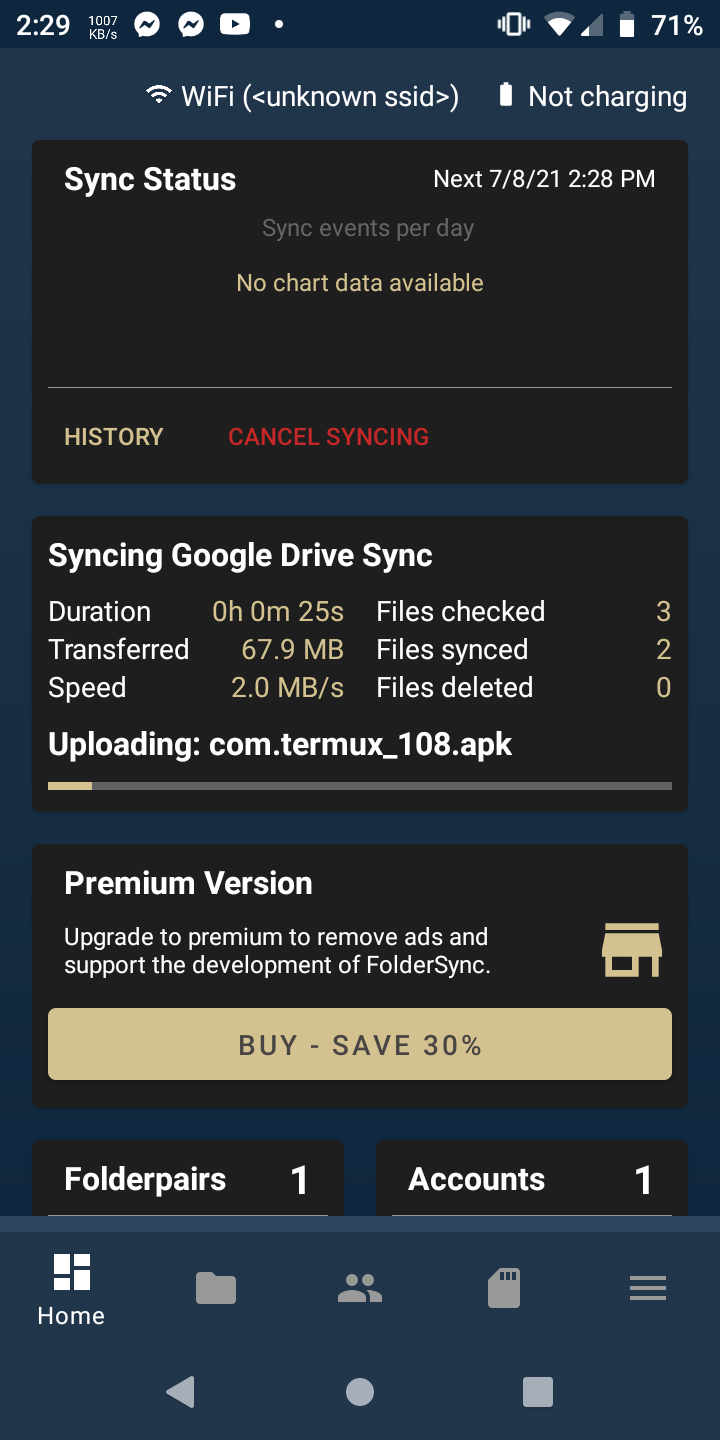This is a screenshot of a smartphone display, showing various UI elements and notifications:

- **Top Bar:**
  - **Left Side:** The current time is displayed in white text as "2:29." Next to the time, there are several notification icons, including two speech bubbles likely representing WhatsApp, a white YouTube icon, and a white dot.
  - **Right Side:** The battery status shows 71% with an accompanying battery icon, a signal icon indicating less than half signal strength, and a Wi-Fi signal icon indicating slightly less than full strength.

- **Wi-Fi and Battery Status:** Below the top bar, white text reads "Wi-Fi Unknown SSID" and there is a battery icon with "Not Charging" displayed next to it.

- **Sync Status:** There is a gray rectangle that indicates "Sync Status." At the top left of this rectangle, in red text, it reads "Cancel Syncing."

- **Sync Progress:** Below the "Sync Status" box, there is another gray rectangle displaying a progress bar for "Syncing Google Drive Sync." The progress bar is tan in color and appears to be between 5 to 10 percent complete.

- **Premium Version Offer:** Further down, there is a gray box with the text "Premium Version" in white. Inside this box, there is a tan button that reads "Save 30%."

Overall, this screenshot captures the phone's notification and syncing status, along with a promotional offer for a premium service.